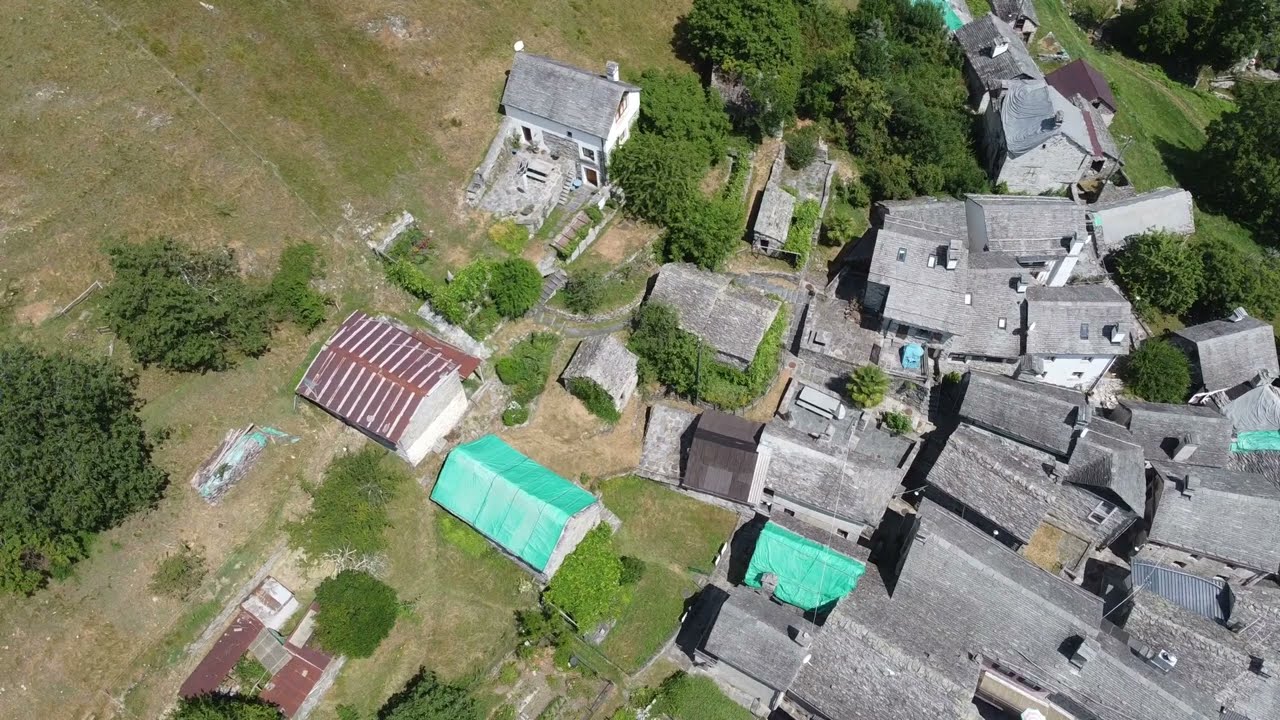This aerial drone photograph, presented in landscape orientation and depicting a high-altitude viewpoint, captures a tight cluster of houses predominantly settled on the right side of the image. These houses feature gray shingle roofs, positioned incredibly close to each other with almost no space for parking, creating a densely packed appearance. On the left-hand side of the image, there is a range of distinctive structures: a small house with a bright aqua-colored roof, and nearby, another with a red tin roof adorned with white stripes. Further to the left is a white and gray house with a gray triangular roof, leading into a green pastured area with rising hills, decorated with green bushes and trees. The upper portions of the photograph showcase clusters of round, green trees that frame the area, with the top right corner revealing a hill descending to the right side, also covered in green grass and trees. The photograph, characterized by its realism and farm-style housing architecture, highlights the contrast between the densely packed residential zone and the sprawling, green natural landscape that encompasses it.